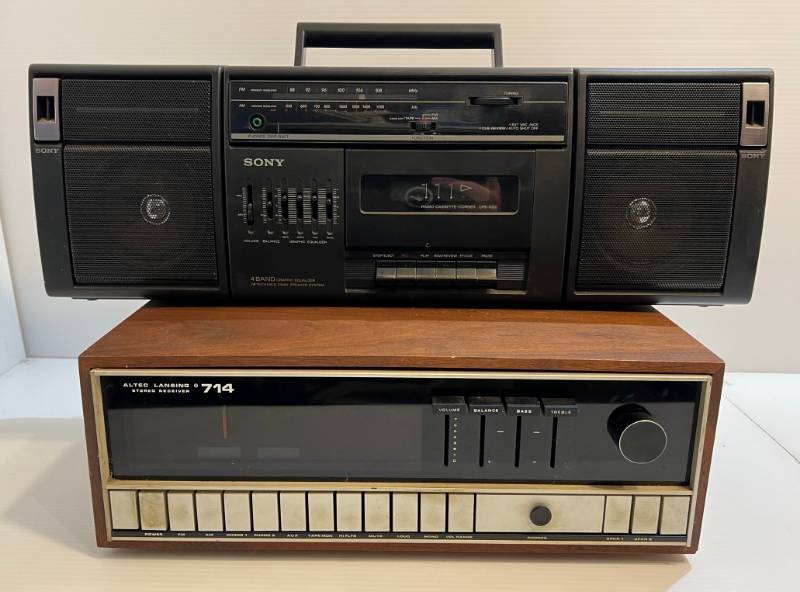This highly detailed, horizontal photograph captures a scene in an all-white room, featuring vintage music equipment in a stark, minimalist setting. Dominating the upper portion of the image is a black Sony portable cassette player, recognizable as a small boombox, complete with a handle at the top. This classic piece, spanning wide horizontally, features two detachable speakers on either side of a central cassette deck, an analog radio tuner, and several adjustable dials and an inline equalizer adjacent to the tape deck. Below the Sony boombox sits a wooden, retro-styled Altec Lansing 714 stereo receiver or amplifier from the 1970s. This device, encased in a wood finish, displays an array of off-white pushbuttons, four black sliders, a black knob, and a black button for various sound adjustments, channel outputs, and effects. The Altec Lansing unit’s cream and wood palette contrasts with the Sony's predominantly black design accented with silver highlights. Together, these historical stereos evoke a sense of nostalgia against the pure white backdrop, emphasizing their vintage charm and functional details.